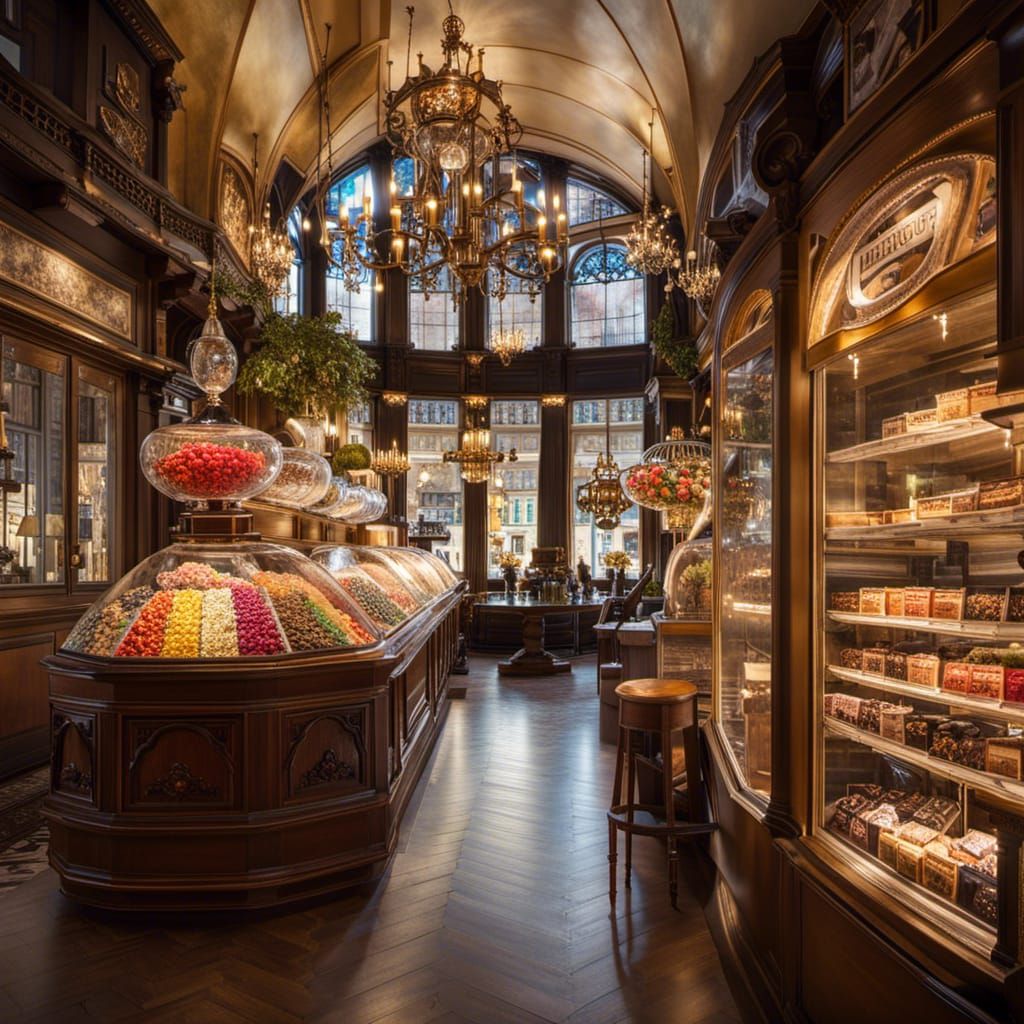The image depicts an intricate and beautifully detailed candy shop situated in a bustling city. The shop exudes an old-fashioned charm, characterized by an elegant arched ceiling adorned with multiple chandeliers, including a prominent large one in the center that appears to be a vintage brown fixture with candles. The floor is shiny and wooden, adding to the antique aesthetic.

Along the left side of the shop, there is a sizable glass display case with a wooden, intricately carved base, filled to the brim with multicolored candies. Atop the case sits a glass bowl brimming with more sweets. On the right, shelves with glass doors showcase an array of chocolates, candies, and other items for sale.

Towards the back, a spacious seating area beneath high ceilings is illuminated by additional chandeliers, and large windows offer a view of the bustling cityscape outside. The central area of the shop features various glass compartments, each sectioned off to display different assortments of foods and candies, enhancing the shop’s inviting and organized appearance. The overall ambiance is warm and inviting, with rich wooden tones and the soft glow of chandeliers providing a nostalgic experience for visitors.